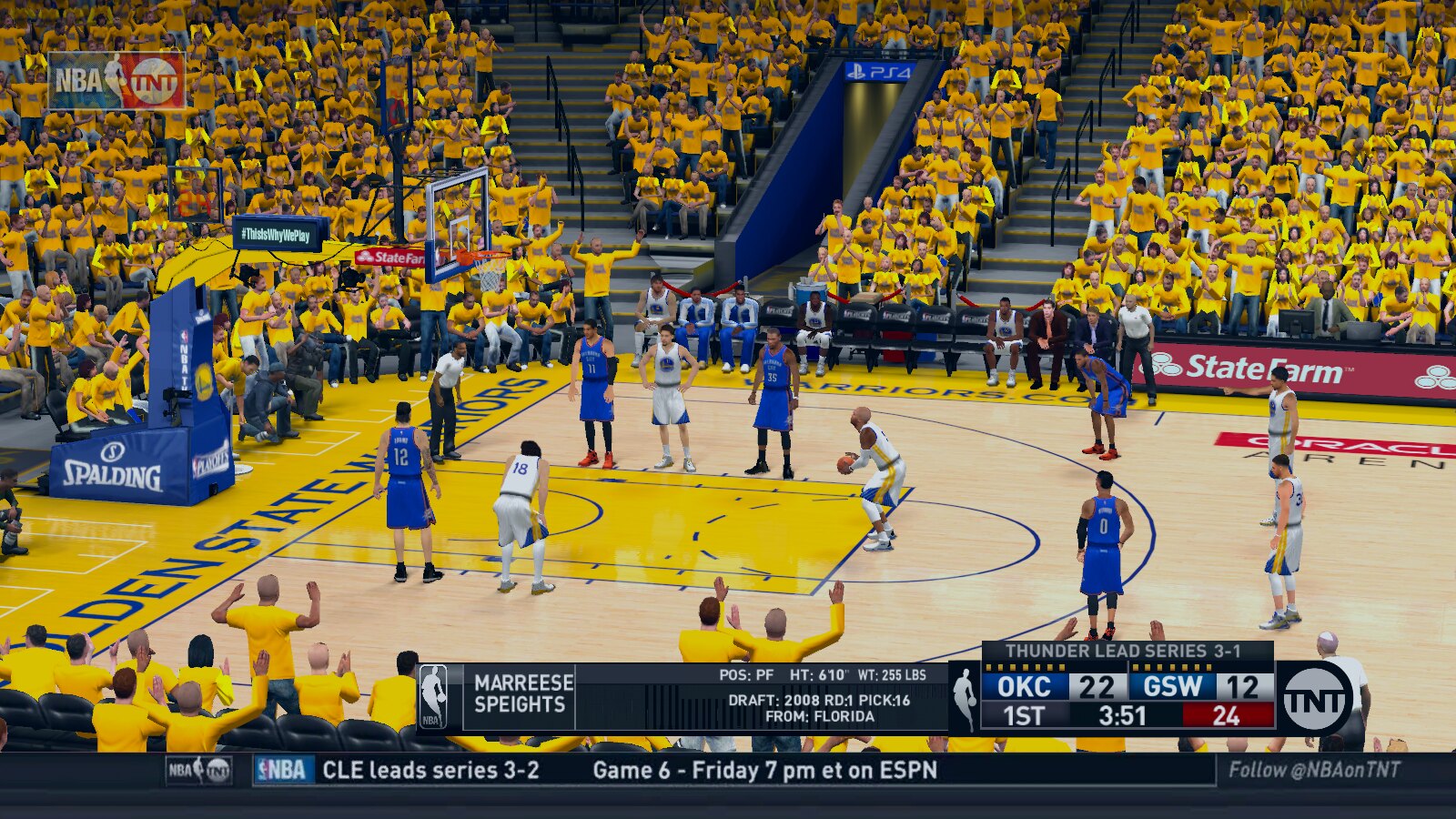The image captures a moment from an NBA playoff game between the Oklahoma City Thunder (OKC) and the Golden State Warriors, broadcasted on TNT. The scoreboard reveals OKC leading 22-12 in the first quarter, with 3 minutes and 51 seconds left and 24 seconds on the shot clock. OKC leads the series 3-1. In the upper left corner, there is the NBA logo alongside the TNT logo. The scene shows Maurice Spates of the Golden State Warriors, positioned at the foul line, with detailed stats displayed: Drafted in 2008, Round 1, Pick 16 from Florida, standing 6'10" and weighing 255 lbs. His information appears in white text on a dark gray background. The court is predominantly tan, with yellow accents on the edges, and the crowd is prominently dressed in yellow, indicating strong support for the Warriors. Blue jerseys dominate the foul line, indicating the presence of the Thunder players. This vivid snapshot encapsulates the intense atmosphere of a high-stakes playoff game in a vibrant stadium setting.